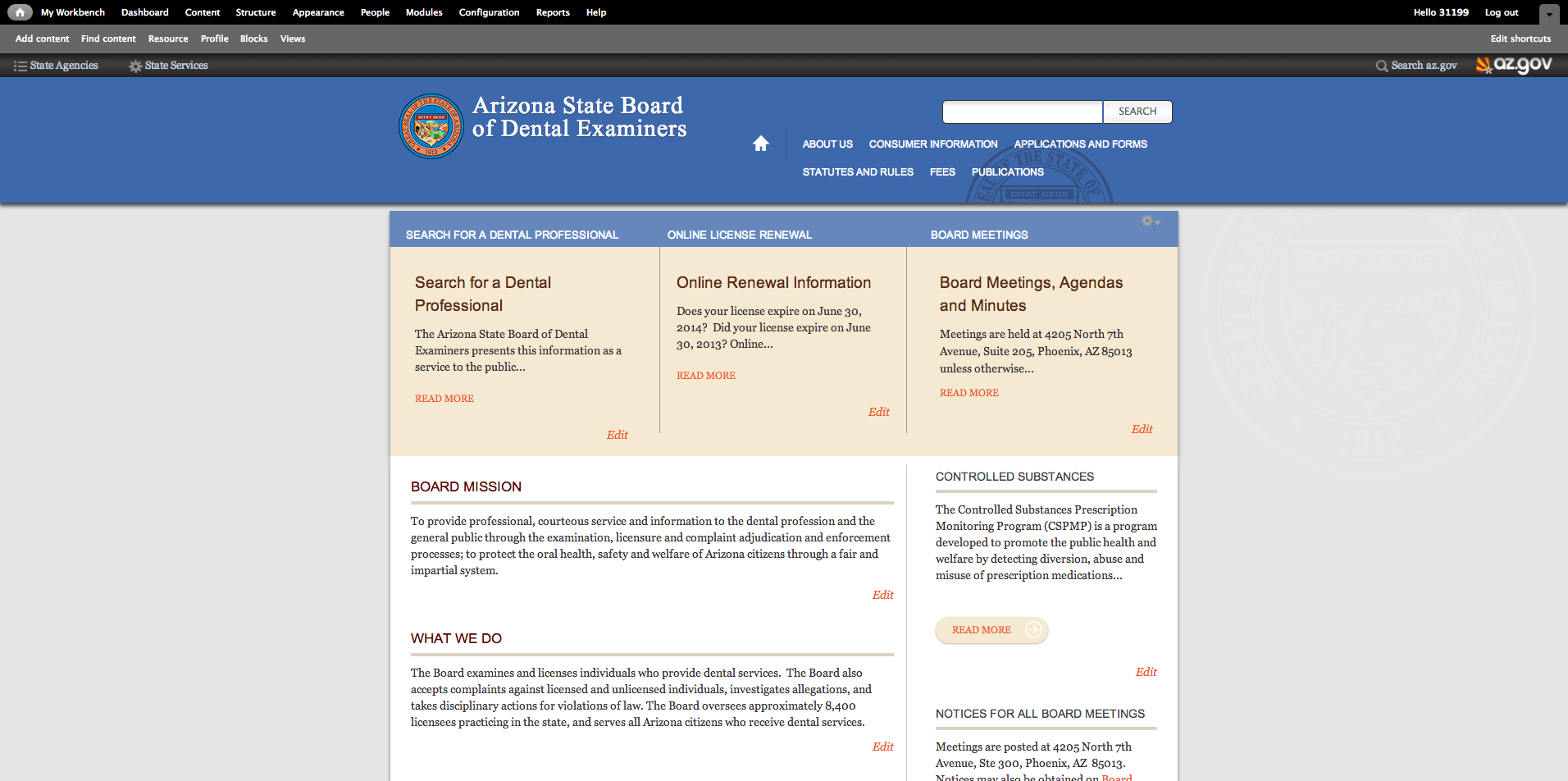This is a landscape-oriented image of the Arizona State Board of Dental Examiners website, showcasing various navigational elements and informational sections. At the top of the webpage is a long, rectangular black border with white text that includes words and links such as "People," "Reports," "Help," and "Lockout," although the font is somewhat indistinct. Below this is another long, rectangular gray border featuring links for "Add Content," "Find Content," "Resources," and additional options that are not entirely legible.

Further down, a darker gray bar presents a bullet-point menu with links labeled "State Agenda," an icon resembling a typing gear followed by unreadable text, "searchaz.gov," and the "az.gov" logo paired with the Arizona state flag.

Positioned below this section is a blue border adorned with the seal of the Arizona State Board of Dental Examiners, alongside a search box for user convenience.

At the bottom of the image, the website features a long, rectangular gray background area which includes a pop-up box. This box is outlined with a blue border and white lettering at the top and has a pink, rectangular background beneath it that displays headers designed to assist users in locating dental information. The section also contains a white box detailing the board’s mission and the services it provides.